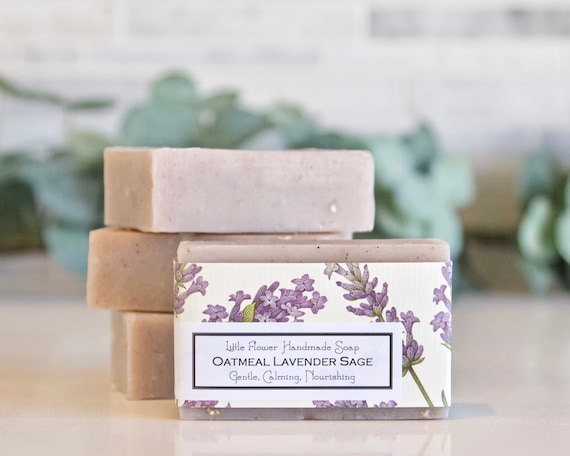The image depicts a sophisticated product display of four bars of soap, ideal for a high-end Instagram post or a bath and beauty store advertisement. Three of the bars are artfully stacked on a pristine, off-white marble surface, while a fourth bar stands upright in the foreground, showcasing its elegant label. The label reads, "Oatmeal Lavender Sage Little Flower Handmade Soap" and touts its gentle, calming, and nourishing qualities. The soap itself is a very light lavender color, complementing the lavender-themed white and purple packaging adorned with delicate drawings of lavender sprigs. The background is a soft blur, hinting at the presence of plants and possibly a kitchen counter backsplash, adding a touch of natural simplicity without detracting from the focus on the meticulously displayed soaps. The overall presentation evokes a sense of refined luxury, akin to products you'd find at Williams Sonoma.